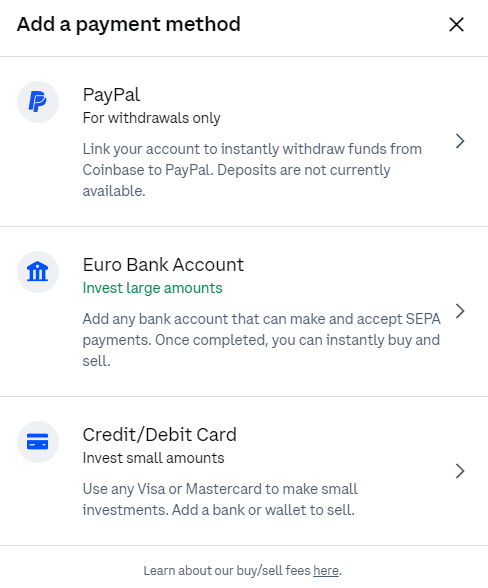The image appears to be a detailed screenshot of a segment from either a mobile app or a website page dedicated to adding payment methods. At the top-left corner, in bold black text, is the title "Add a Payment Method," juxtaposed with a close icon (X) on the top-right side. The first section features a large blue "P" resembling the PayPal logo, accompanied by a description stating "PayPal for withdrawals only. Link your account to instantly withdraw funds from Coinbase to PayPal. Deposits are not currently available."

Below this, a blue icon resembling a museum building introduces the "Euro Bank Account" option. The associated text highlights the purpose: "Invest large amounts. Add any bank account that can make and accept SEPA payments. Once completed, you can instantly buy and sell."

Following this, there is another blue icon, this time representing a credit card. The corresponding information specifies "Credit/Debit Card. Invest small amounts. Use any Visa or MasterCard to make small investments. Add a bank or wallet to sell."

At the very bottom, written in a slightly smaller font, is an informational link: "Learn about our buy/sell fees here." Each payment method entry contains an arrow icon, suggesting the user can click for more details, and these entries are organized vertically in a column format.